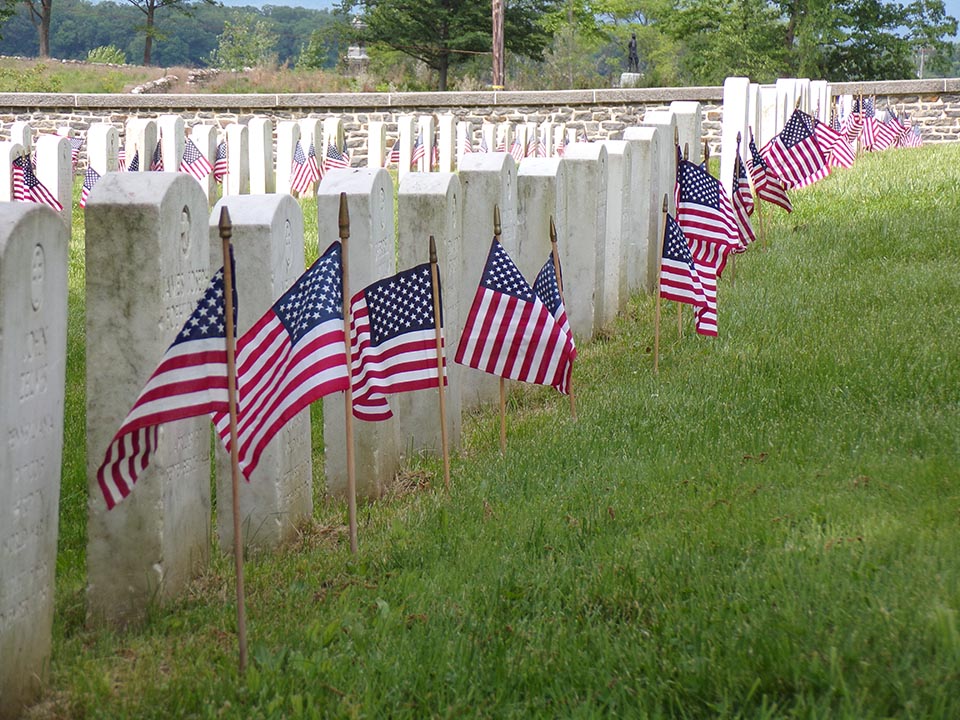The photograph captures a solemn scene at what appears to be a military veteran cemetery. Neatly aligned gravestones, all identical in shape, with arched tops carved from gray stone, extend from the bottom left corner to the middle and top right of the image. Each gravestone is adorned with a medium-sized American flag, planted on a wooden stake in front. The flags' red, white, and blue colors stand out vividly against the lush, green grass, which is tall and well-maintained. In the background, there's a brick retaining wall composed of gray bricks layered with white cement. Beyond the wall, a telephone pole and trees filled with summer foliage complete the serene setting. The overall atmosphere is one of respectful remembrance, honoring the fallen heroes resting in this meticulously cared-for space.